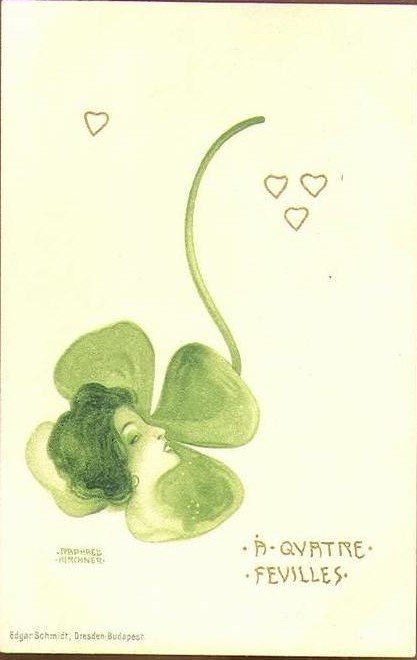This image is a detailed painting resembling a postcard, featuring a prominent four-leaf clover located towards the bottom left-center of the composition. In the center of the clover, painted in green, is the face of a woman with dark hair styled up, her neck extending into the fourth leaf. Her raised eyebrows and suggestive gaze are directed towards the lower part of the image. The right side of her face, where the nose is facing, blends slightly into the adjacent leaf, and her eye is depicted without a visible pupil.

The clover, inverted with its stem curving upwards, positions the stem at the top of the image. Surrounding the stem are heart shapes: three hearts outlined in a triangular arrangement on the right, and a single outlined heart to the left. The leaves of the clover themselves are also slightly heart-shaped, enhancing the thematic consistency.

At the bottom left corner of the postcard, the artist's signature reads "Edgar Schmidt, Dresden, Budapest," while additional text, possibly reading "Akatlefe," appears to the right and lower side of the clover. The background is a clean white, providing a stark contrast to the green of the clover and the woman's face, making them stand out prominently.